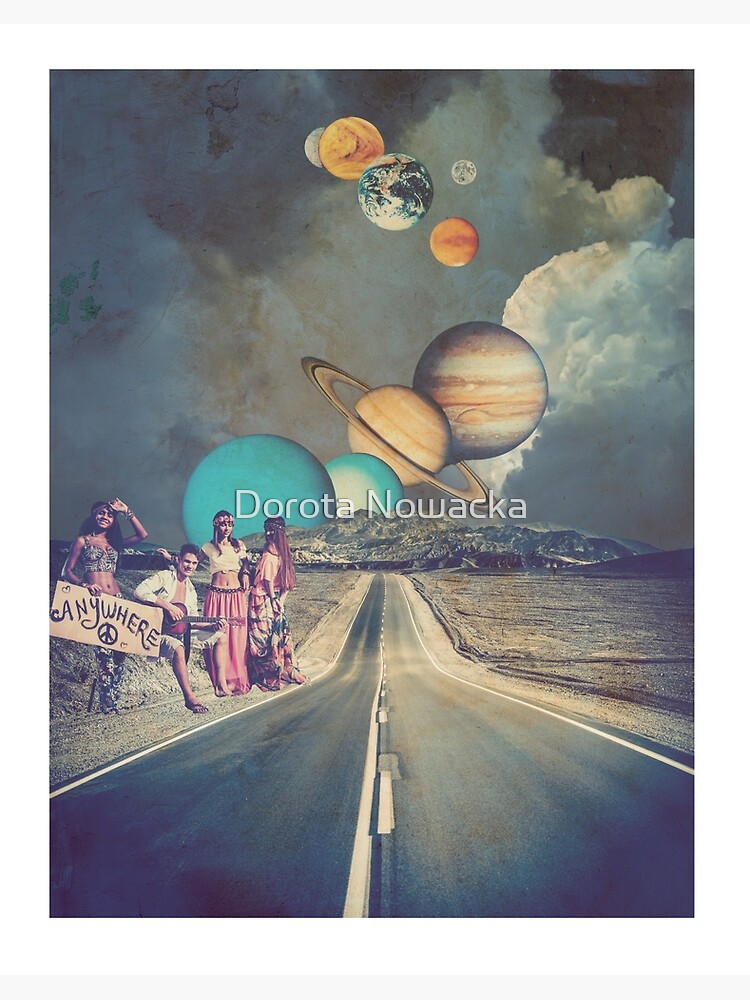This digitally created artwork, likely a poster or card, presents a surreal and imaginative scene of our solar system. Dominated by a central blacktop highway that begins at the bottom and extends into the horizon, the road vanishes into the distance, leading the eye up toward a sky filled with planets. The bottom half of the image shows four young people, possibly festival-goers, standing on the side of the road in a barren desert. One holds a sign that reads "anywhere" with a peace symbol, suggesting a willingness to explore the solar system.

The top half of the image features a layered sky background with dark cumulus clouds and an array of planets, including Earth, Saturn, Jupiter, Uranus, and Mars, among others. These planetary bodies do not adhere to realistic proportions but add to the fantastical essence of the artwork as they rise beyond a distant mountain on the horizon. 

In the center of the image, prominently displayed in thin white lettering, is the name "Dorota Nowaka," presumably the artist behind this intricate design. This creative piece masterfully combines photographic elements with graphic illustrations, emphasizing the whimsical journey of the young adventurers as they embark on an interplanetary adventure.